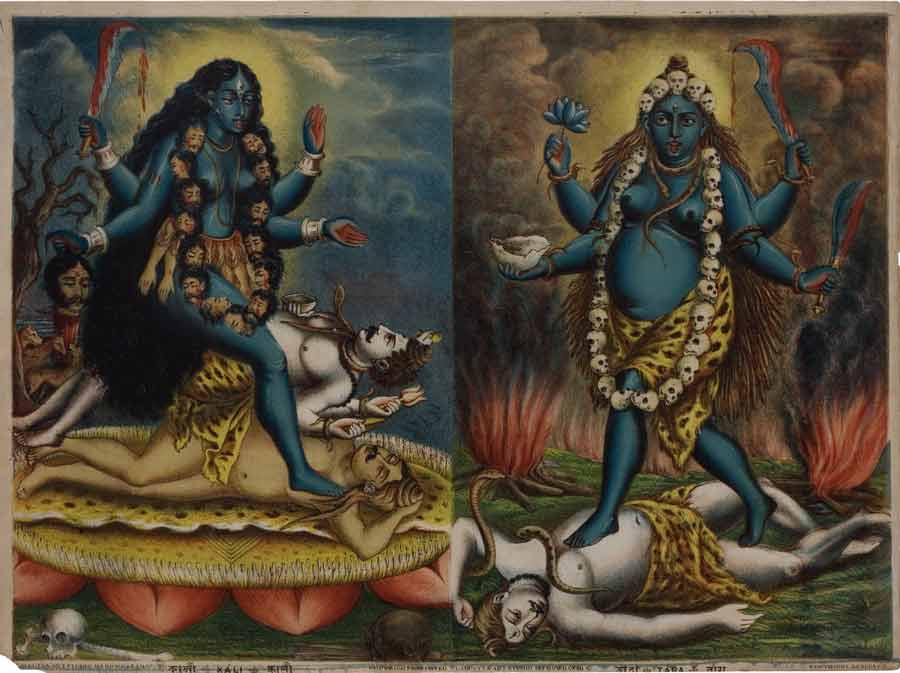This image features two adjacent paintings that appear to be inspired by Hindu art, each depicting a blue-skinned, four-armed female deity with distinct attributes and actions. 

In the left painting, the female figure is adorned with a necklace made up of severed human heads, which extends down to her knees. She has flowing long black hair and holds a bloody knife in one of her right hands while clutching a severed head in the other right hand. Her left hands hold different objects, including another machete and a flower. She stands with one foot on a body that lies prone on a yellow carpet decorated with pink petals. Nearby, a skull and a skeleton add to the eerie atmosphere.

The right painting similarly features a blue, four-armed female deity, but with subtle differences. She wears a necklace of skulls and heads, along with a headpiece adorned with the same macabre elements. Her upper right hand holds part of a skull, while her other right hand holds a blue lotus flower. In her left hands, she carries a bloody knife and a bowl. Like the figure in the first painting, she is stepping on a person, who in this case is covered in snakes. Both images are set against backdrops with a blue sky, adding to the unorthodox and mystical style of the art.